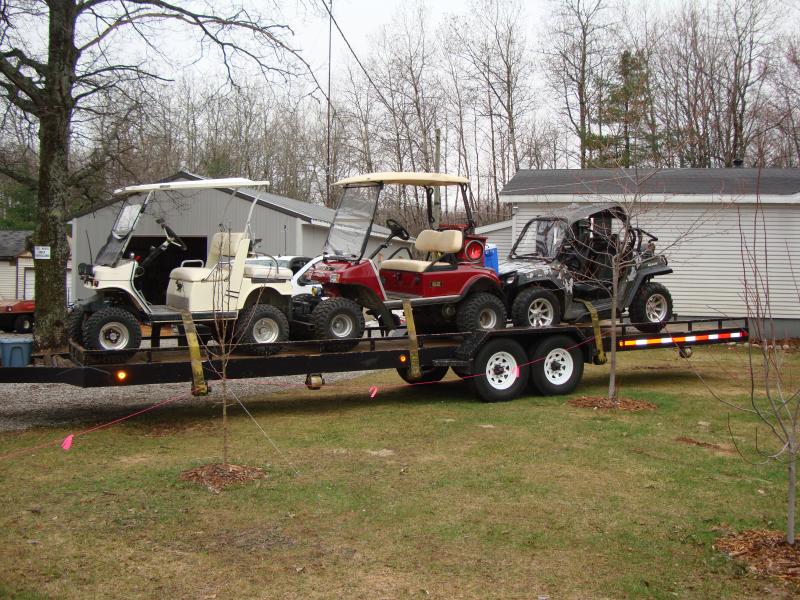In this photograph, a lengthy dark brown trailer hitch with black tires and white rims is seen in the foreground, laden with three vehicles. At the front of the trailer, there is a white golf cart with matching white seats and black wheels. Behind it, the second vehicle is a red golf cart featuring off-white seats and a roof cover, while the third and final vehicle is a greyish small car or dune buggy with a black top. The three vehicles are securely strapped with thick, tannish-brown straps.

The trailer, parked on light green grass, is situated near a series of buildings with grey roofs and grey siding. The scene appears to be a backyard setting, featuring houses and a possible warehouse with an open large door revealing a dark interior. Notably, in the background, sparse leafless trees and a single evergreen punctuate the landscape, and newly planted young trees with mulch at their base are interspersed across the lawn. A safety reflector adorns the back of the trailer. The sky overhead is grey, adding to the muted, wintry atmosphere of the scene.